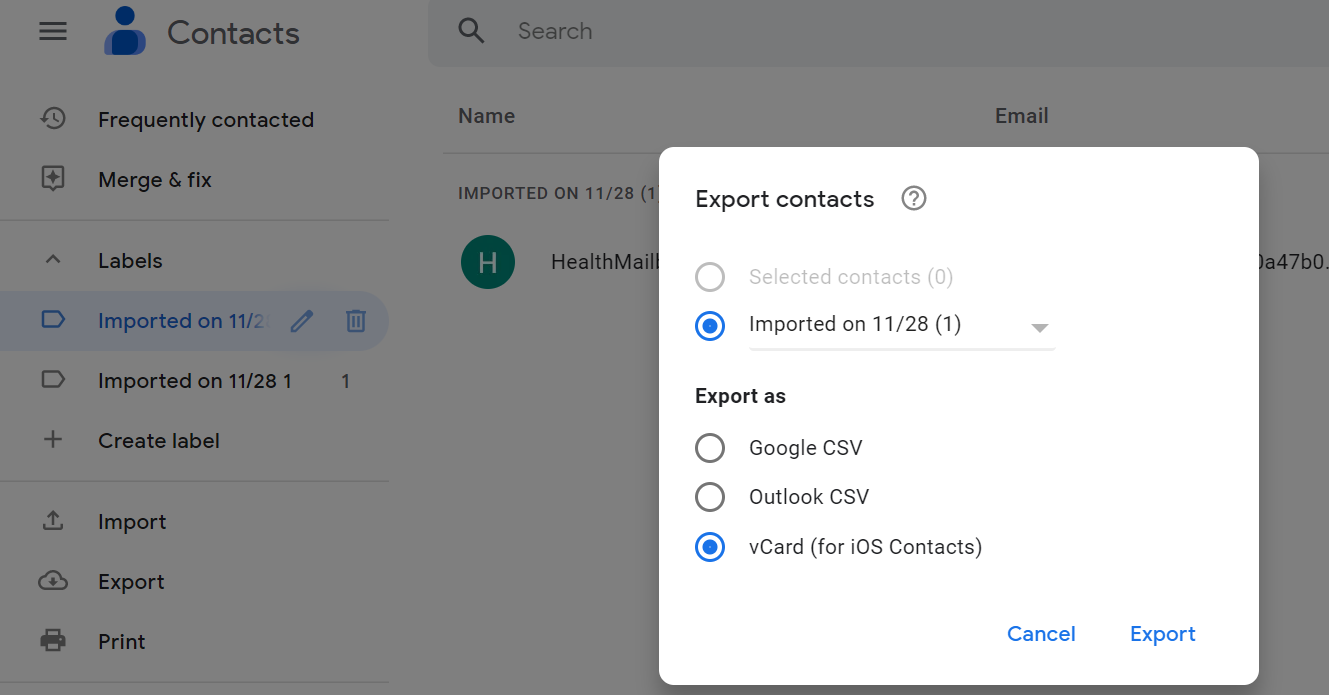The image depicts a user interface screen related to managing contacts. There is a prominent gray rectangle in the foreground, partially overlaid by an illuminated white square. The background of the rectangle features the word "Contacts" faintly visible due to the shading effect.

Within the white square on top of the gray rectangle, the heading reads "Export contacts," accompanied by a question mark inside a circle. Below this heading, the screen shows "Selected contacts: 0" followed by "Imported on 11/28" with a number "1" in parentheses next to a blue dot. 

Following, there are export options listed: "Google CSV," "Outlook CSV," and "vCard for iOS contacts," with the circle next to "vCard for iOS contacts" highlighted in blue. 

The bottom right corner of the square features two buttons: "Cancel" and "Export."

In the shaded background, a vertical list reads: "Frequently contacted", "Merge and fix", "Labels", "Import", "Export", and "Print". On a subsequent row, a search button appears, followed by column headers "Name" in the middle and "Email" to the right. Additionally, there is a green button with a white "H" icon labeled "Health Mail," partially obscured by the white square.